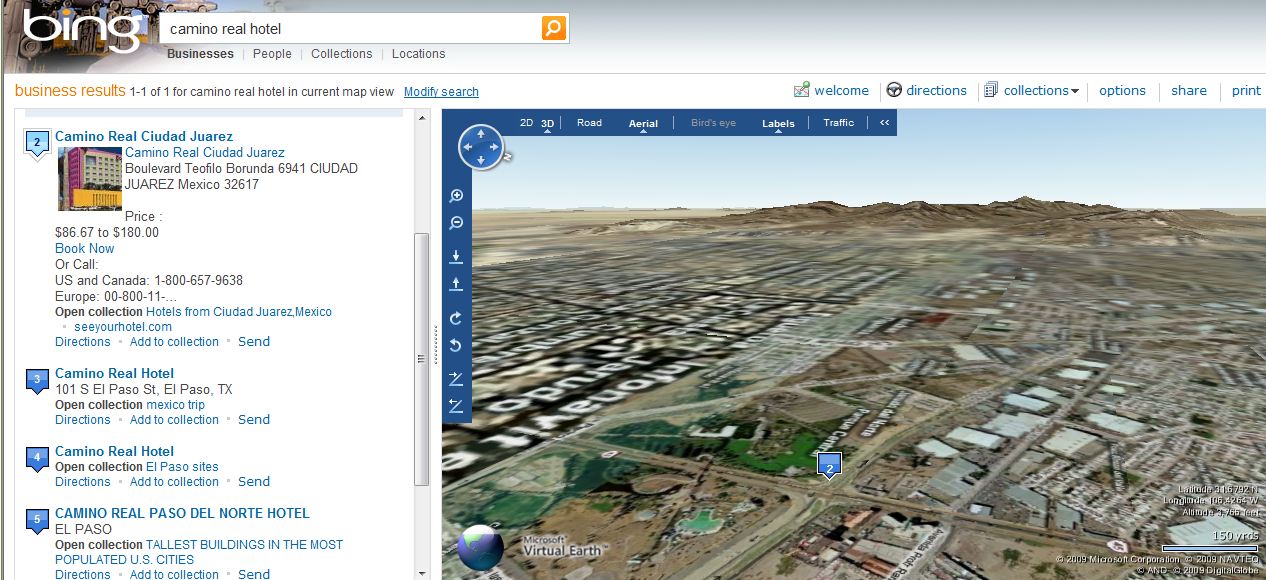The image captures a screenshot of a Bing search results page. At the top of the screen, the search query "Camino Real Hotel" is clearly entered. Below this, a satellite map view dominates the main section, zoomed in on the center of an intersection. To the left of the map are listed business results related to the search term.

The first result highlights "Camino Real Ciudad Juarez" in Juarez, Mexico, displaying a price range of $86.67 to $180. Options to "Book Now" or call are provided, with distinct phone numbers for the U.S. and Canada, as well as Europe. The next listing shows "Camino Real Hotel" in El Paso, Texas. Additional entries include another "Camino Real Hotel" in El Paso and "Camino Real Paso Del Norte Hotel" also in El Paso.